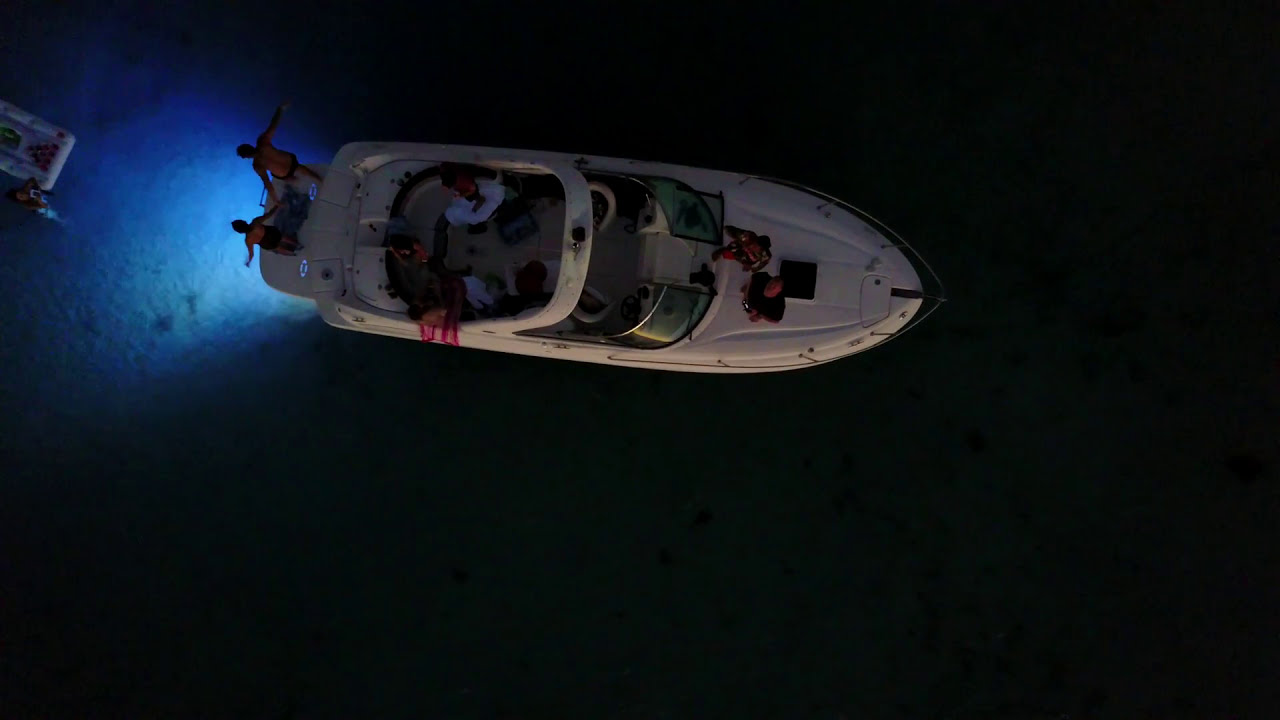This is a nighttime aerial photograph of a white fiberglass boat on dark water, illuminated by a light, likely coming from the boat, casting a blue glow on the water near the vessel. The boat is facing to the right of the image, and we can see several people on board. At the front of the boat, also referred to as the bow, a couple of individuals are standing and looking upwards. In the back of the boat, two more people are either in darkness or not clearly visible, possibly adding up to three individuals. On the rear of the boat, specifically on the diving step, two people in bathing suits are holding hands and appear to be preparing to jump into the illuminated water below. Additionally, a small floating platform, which might be a rubber raft, is positioned a short distance away from the boat, with a person clinging to its side. The boat features tinted windshields on either side and has a long bow, enhancing the overall silhouette.